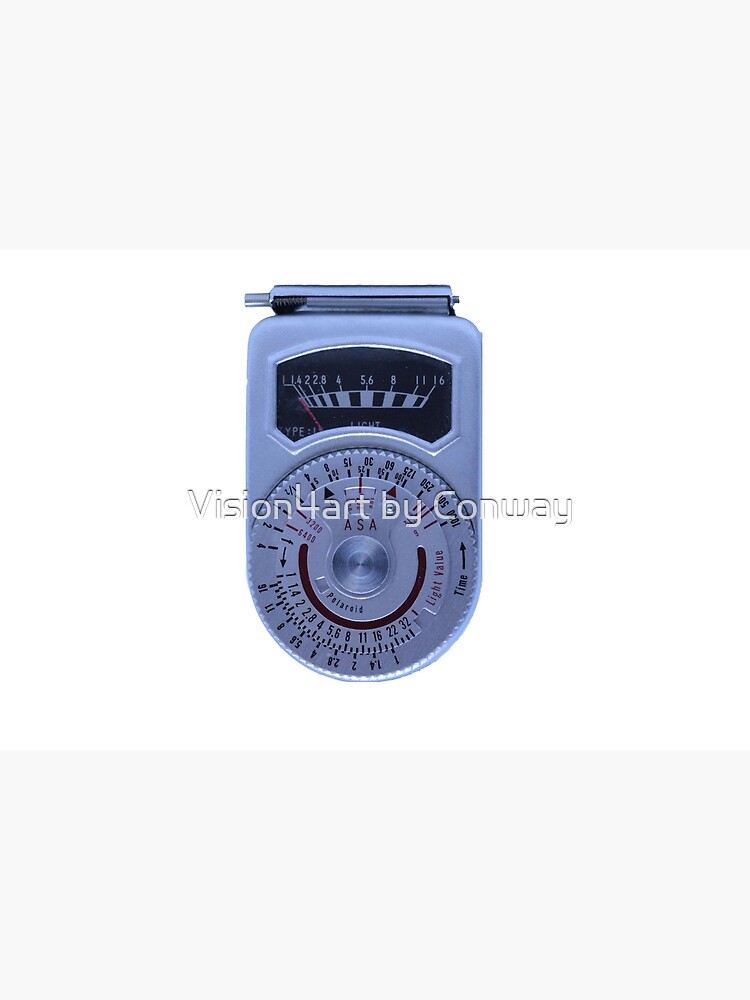The image depicts a blue-tinted, wall-mountable device, possibly a thermostat or a meter, set against a background featuring two light-gray rectangles on the top and bottom, with a white section in the center. The device prominently displays the text "Vision 4 Art by Conway" in a central white text. It features a circular dial adorned with red numbers and arrows, used for adjustments, alongside several technical terms and measurements including ASA, light value, time, and Polaroid. Above the dial is an analog display with a red needle pointing to various numbers such as 4, 2, 22, 8, 4, 5.68, 11, and 16. Additional text on the display includes partially visible words like "type", "plus one", and "LIGHT". The screen at the top of the device shows some blue font text against a black background, though parts of it are difficult to read.